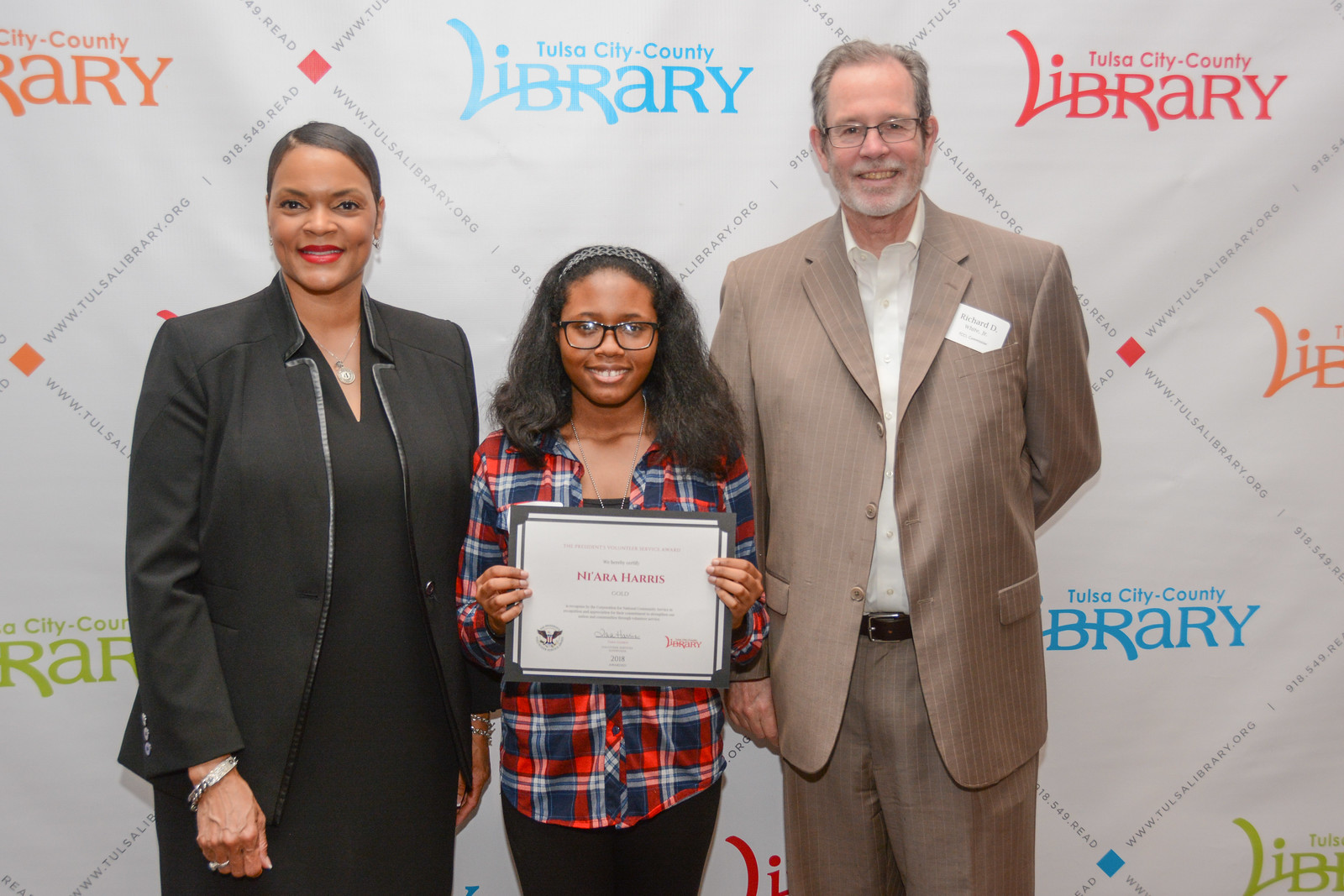In the image, three individuals are posed in front of a white wall adorned with a pattern created from black font that reads "www.tulsalibrary.org" along with various phone numbers, forming diamond shapes. Inside the diamonds, the text "Tulsa City County Library" is repeated in alternating colors of red, blue, and orange. 

At the center is a young African American girl named Nayara Harris, identifiable from the certificate she is holding. Nayara sports shoulder-length, slightly poofy, straightened hair held back by a headband, and wears black-rimmed glasses. She is dressed in a red, white, and blue plaid shirt and black pants.

To Nayara's left stands an African American woman, slightly older, with slicked-down hair pulled back behind her head. She dons bright red lipstick and is dressed in a black V-neck dress topped with a black coat, complemented by silver earrings.

On Nayara's right is an elderly Caucasian man with gray hair, a white beard and mustache, and glasses. He is clad in a tan pinstripe suit jacket and pants, paired with a white collared shirt. All three are looking toward the camera, seemingly at an award ceremony, with the wall prominently displaying the Tulsa City County Library branding behind them.